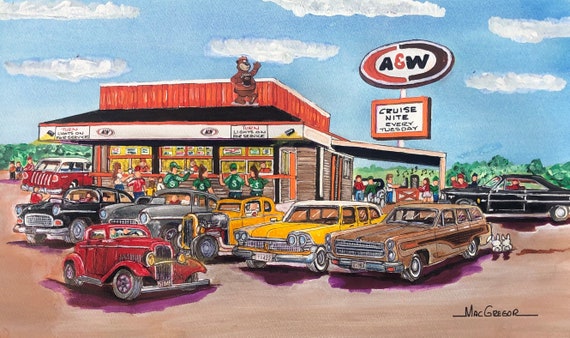This vibrant painting, signed "McGregor" in the lower right corner, captures a lively 1950s A&W drive-in scene, bustling with activity. Dominating the foreground is a striking red hot rod, a modified Model T. Close by, a distinctive bright yellow station wagon resembling a taxicab with a white roof adds to the nostalgic charm. A brown station wagon with wood paneling and a sleek black '55 Chevy are also prominently displayed among the array of classic cars. Atop the drive-in, the iconic A&W logo, featuring the distinctive orange 'C' and reverse black 'C', is prominently displayed. Below it, a sign announces "Cruise Night every Tuesday," (mistakenly remembered as Thursday in one description) attracting a crowd of car enthusiasts. Adding character, a whimsical bear figure completes the nostalgic ambiance. The painting's colorful palette and detailed portrayal make this scene both inviting and richly evocative of a bygone era.